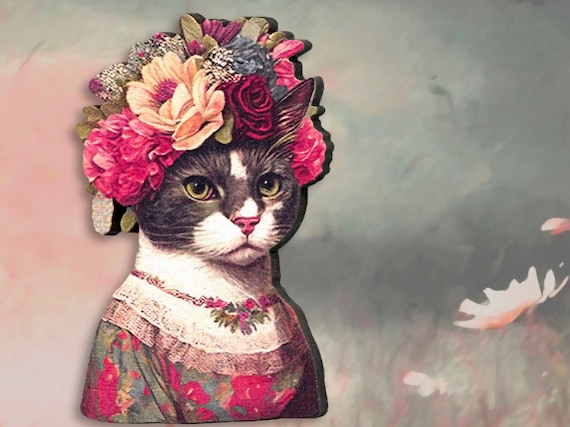The image is a horizontally-oriented rectangle depicting a Victorian-style portrait of a tabby cat with distinct white facial markings. This short-haired cat, primarily dark gray with a white blaze between its yellowish-green eyes, sports a white snout and a white neck. The cat is anthropomorphized, dressed in a floral Victorian dress accented with a high, white lace collar, around which some flowers are delicately embroidered. Sitting upright, the cat's body is visible from the chest up, without showing its paws or legs.

Adorning the cat's head is a lavish garland composed of diverse flowers, including red roses, pink chrysanthemums, and various yellow, blue, and green flowers interspersed with greenery. A noteworthy detail is one ear protruding through a gap in the floral crown, while the other ear remains nestled beneath the blooms. The background is an impressionistic blend of muted pink, green, and gray hues, evoking a sense of classic, refined elegance. In the lower right-hand corner, there’s an additional detail of a small, out-of-focus flower or leaf, contributing to the overall soft and subtle aesthetic of the artwork. The cat’s dignified and somewhat striking pose echoes the style of a stately, historical portrait, reminiscent but distinctly Victorian rather than evocative of Frida Kahlo's boldness.